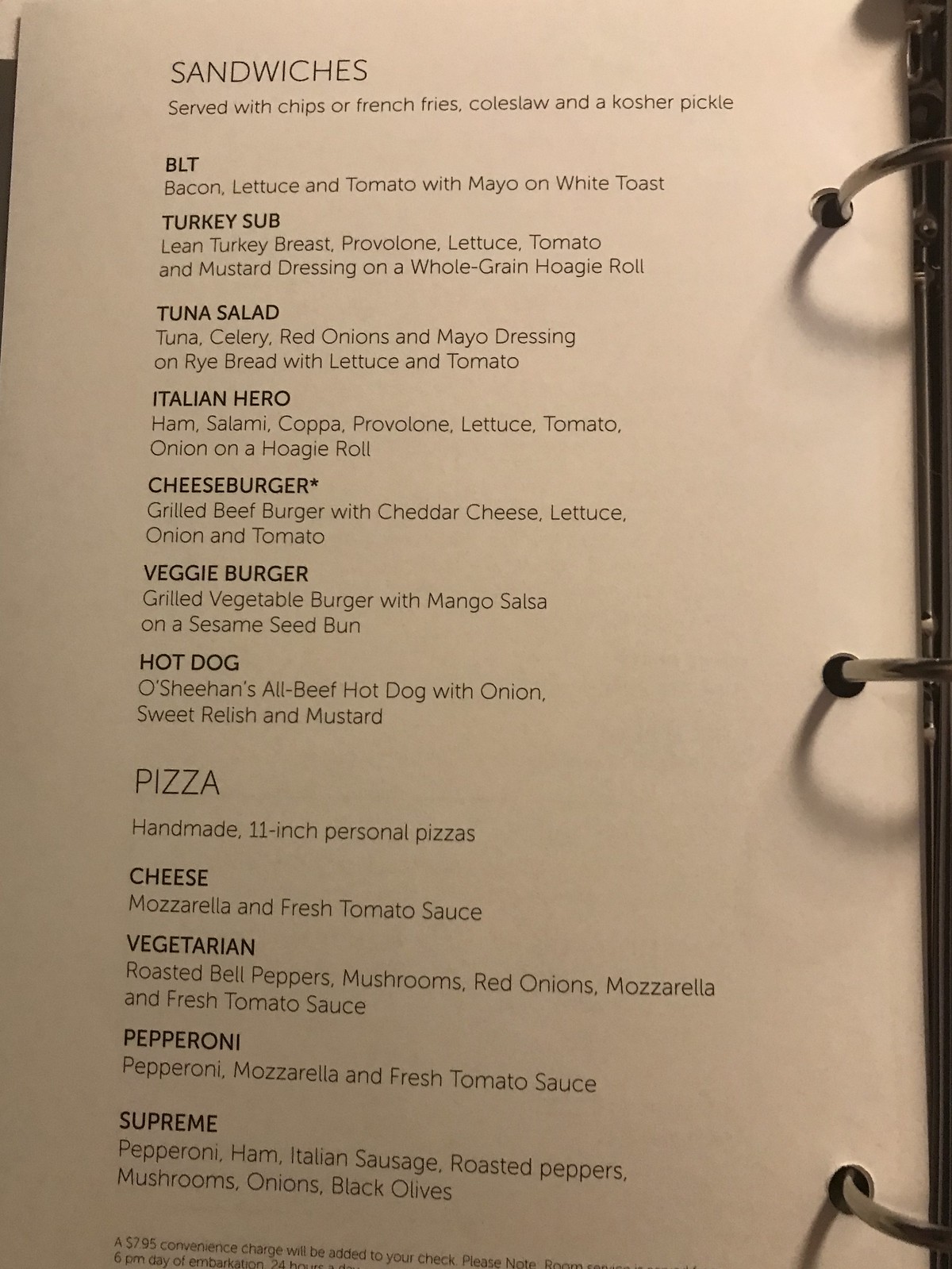The photograph showcases a menu page which is part of a loose-leaf binder. The page itself is a soft pinkish-gray hue, neatly secured by three shiny chrome rings on its right side, each ring punctuating a corresponding hole in the paper. Stainless steel or chrome rods run parallel to the rings, casting subtle shadows on the menu page.

The menu starts with a bold heading in black letters: "Sandwiches." Directly below it, the text reads, "Served with chips or french fries, coleslaw, and a kosher pickle," indicating the accompaniments to the sandwich offerings. Several sandwich options are listed beneath, including Cheeseburger, Veggie Burger, and Hot Dog, though no prices are provided. Further down, another section is dedicated to pizzas, described as "Handmade 11-inch personal pizzas," followed by an array of flavor options. The overall presentation is clean and simple, focusing on the offerings without clutter.